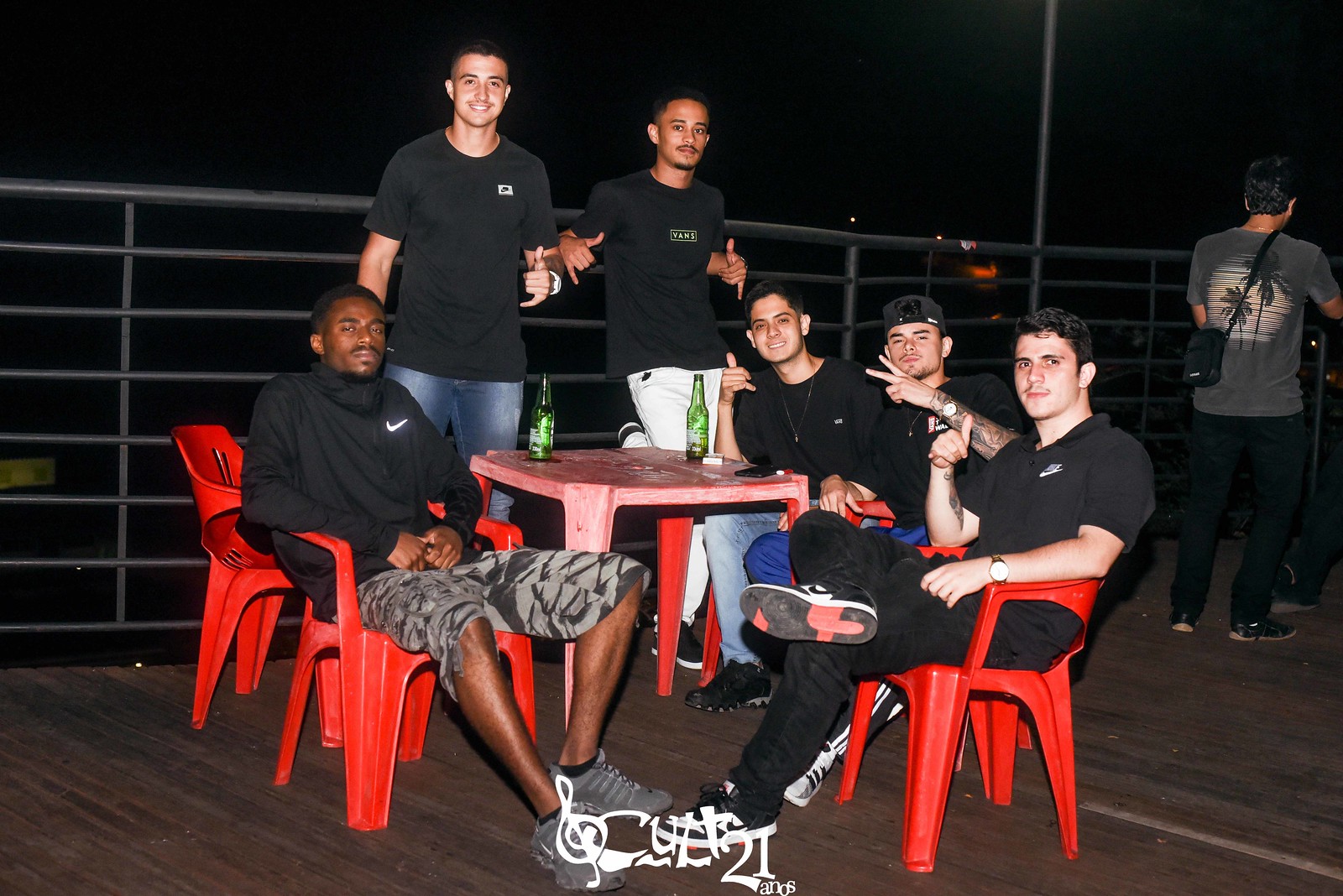The photograph captures a group of young men lounging around a red plastic table on a wooden patio or deck with tall metal railings. The scene appears to be set at night, indicated by the completely black background. Each of the men is wearing black tops, and their attire includes a mix of black pants, blue jeans, and a distinctive pair of gray camouflage shorts paired with a black Nike hoodie featuring a white check mark on the chest. They're seated in matching red plastic lawn chairs. On the table, there are two green glass bottles, likely beer bottles. The men, who appear to be Hispanic or Middle Eastern and one Black man, are enjoying a casual evening together, their similar attire and relaxed postures suggesting a sense of camaraderie and shared experience.